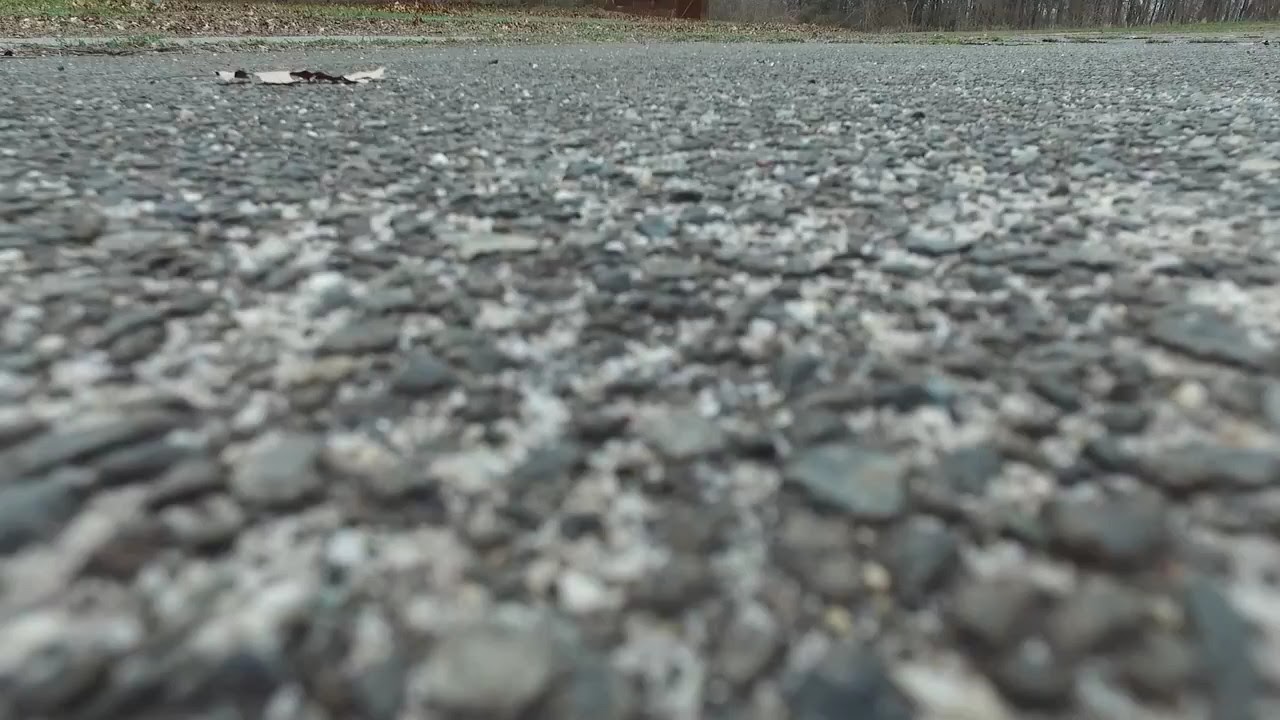This image presents an up-close view of a weathered asphalt surface, predominantly characterized by its gray, bumpy texture interspersed with small, rocky gravel. The ground is dotted with bits of dirt that have naturally settled into the cracks over time. A single grayish-beige leaf rests on the surface, appearing to hover slightly as you can see both above and below it. Captured from a low angle, almost as if taken by someone lying on the ground, the composition emphasizes the asphalt, which occupies about 95% of the frame. In the distance, the scene reveals a curb or sidewalk with adjacent grass and glimpses of trees without leaves. Additionally, there's a reflective pool of water on the top right corner that mirrors the surrounding trees, and on the top left, patches of dirt and grass encroach upon the asphalt. The image is set in daylight, providing a clear, detailed representation of both the texture and components on and around the road.